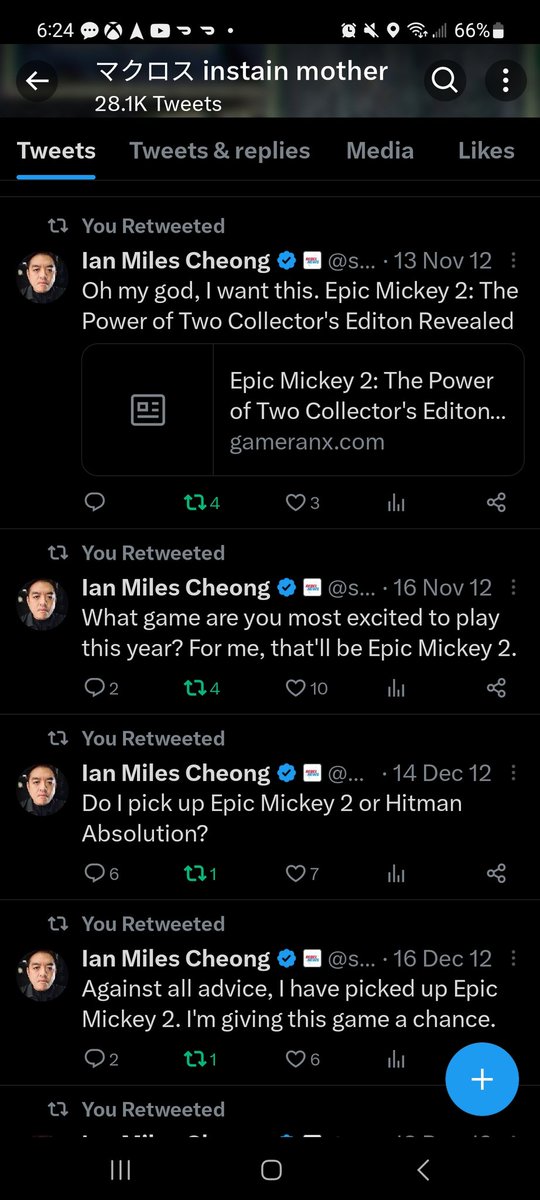Here is a cleaned-up and detailed caption for the described screenshot:

---

This screenshot, taken on a cell phone, captures a Twitter interface where various icons are visible at the top of the screen, including a text bubble, Xbox, YouTube, and DoorDash on the left, and an alarm clock, muted speaker, Wi-Fi, and a battery at 66% on the right. The header displays "INSTAIN MOTHER" with Japanese katakana to the left, translating to "Macross." There is a magnifying glass icon indicating a search, showing "28.1 thousand tweets." 

Below are the navigation tabs for "Tweets," which is currently selected, "Tweets and replies," "Media," and "Likes." The content includes several retweeted posts by Ian Myles Cheong, with the user expressing enthusiasm about "Epic Mickey 2: The Power of Two Collector's Edition." The retweets reveal the user's anticipation for the game and their decisions revolving around it:
- "Oh my god, I want this. Epic Mickey 2, the Power of 2 Collector's Edition revealed."
- "What game are you most excited to play this year? For me, that'll be Epic Mickey 2."
- "Do I pick up Epic Mickey 2 or Hitman Absolution?"
- "Against all advice, I have picked up Epic Mickey 2. I'm giving this game a chance."

---

This detailed caption effectively conveys the content and context of the screenshot.